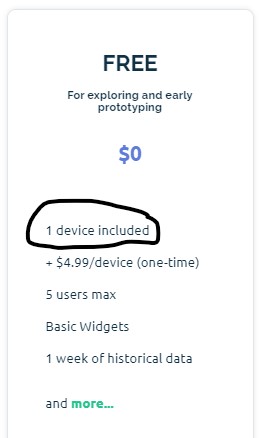The image appears to be a photo of a phone screen displaying a pricing plan with a white background. The information is presented in green and blue text, with various elements aligned in a structured manner. 

- At the top of the screen, the word "FREE" is prominently displayed in large, capitalized green letters and is center-aligned.
- Below "FREE," in much smaller green text, it reads "for exploring and early prototyping," also centered.
- Beneath this description, the price "zero dollars" is presented in blue text, center-aligned.
- Further down, the text shifts to the left, detailing "One device included," which is circled in black.
- Below this, there's more information in green text stating, "plus $4.99 per device one time."
- The next line lists "five users max," followed by "basic widgets," "one week of historical data," and a clickable "more..." link highlighted in bright green.
- The entire content is enclosed in a gray rectangle, though the bottom part of the box appears to be cut off.

Overall, the text outlines the features of a free plan with an option to add more devices for a one-time fee and includes basic functionality, limited user access, and minimal data history.